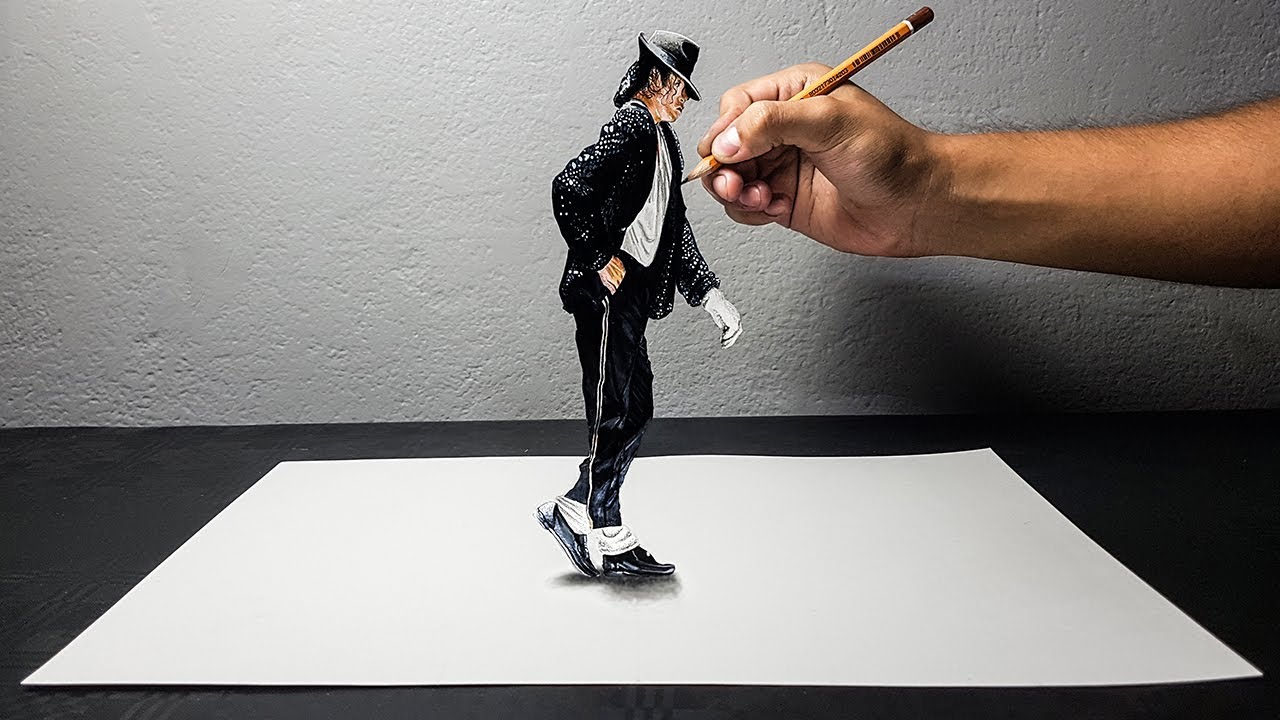The image vividly captures a detailed scene with a small 3D figurine of Michael Jackson as the focal point. Michael Jackson is depicted wearing a sequined black long-sleeved coat, black pants, and black dress shoes adorned with puffy white socks (spats). His signature style is further highlighted by a black hat, long curly black hair, and a single white glove on his left hand, while his right hand is inserted into his pocket. Positioned as though he is about to moonwalk, his figure casts a subtle shadow below his shoes. A noteworthy detail is a hand extending from the right side of the image, holding a pencil poised over the figurine, giving the appearance that it is being sketched onto a white piece of paper that lies flat on a black surface, likely a table. The backdrop consists of a plain white plaster wall, providing a clean and contrasting setting for the vibrant and well-lit scene.